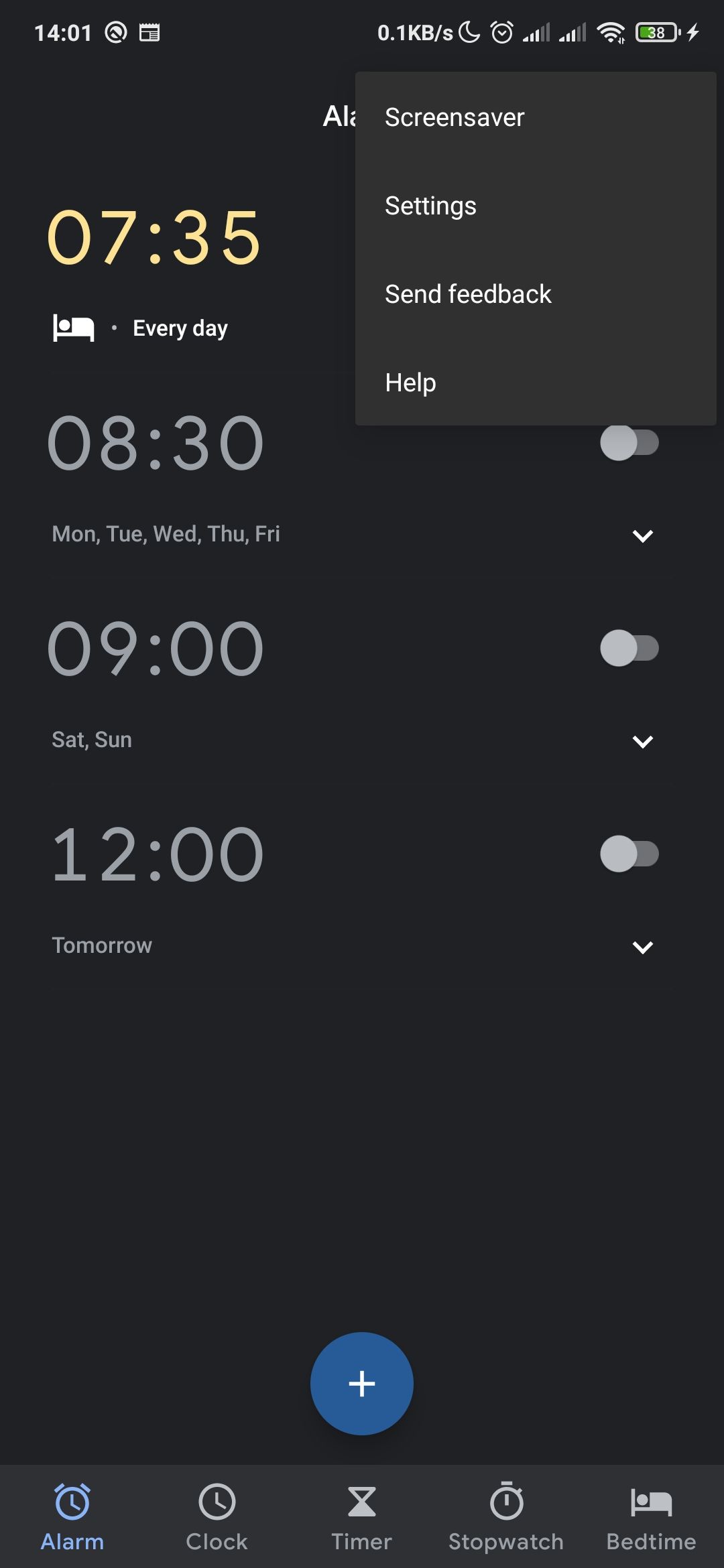A detailed mobile screenshot of an Android device displaying the clock and alarm settings interface. The time shown on the device is 14:01. The status bar at the top includes various icons: a mountain with a circle, likely representing a specific app, a calendar page icon, and an indicator showing data usage at 0.1 kilobytes per second. The device has notifications snoozed and an alarm activated. Two separate cellular networks are visible, both showing three bars of signal strength, alongside a fully connected Wi-Fi signal. The battery is charging and currently at 38%.

In the foreground, there's a dark gray menu pop-up displaying options such as Screen Saver, Settings, Send Feedback, and Help. Below this, the alarm settings are visible. There are multiple alarms configured: 7:35 AM daily, marked with a person in bed icon and currently highlighted; 8:30 AM for Monday through Friday, toggled off; 9:00 AM for Saturday and Sunday, toggled off; and an alarm set for 12:00 (unspecified a.m. or p.m.) for the next day. There is also a blue plus icon available for adding more alarms.

At the bottom of the screen, the interface features an old-style alarm clock icon, highlighted in pale blue against a dark gray-black background. Following this are icons and labels for different tools: a clock, a timer marked with an hourglass, a stopwatch, and a Bedtime setting identified with a person in bed icon. This screenshot highlights the comprehensive alarm management interface on an Android device, though the presence of the Screen Saver and other menu options above it is somewhat unclear.